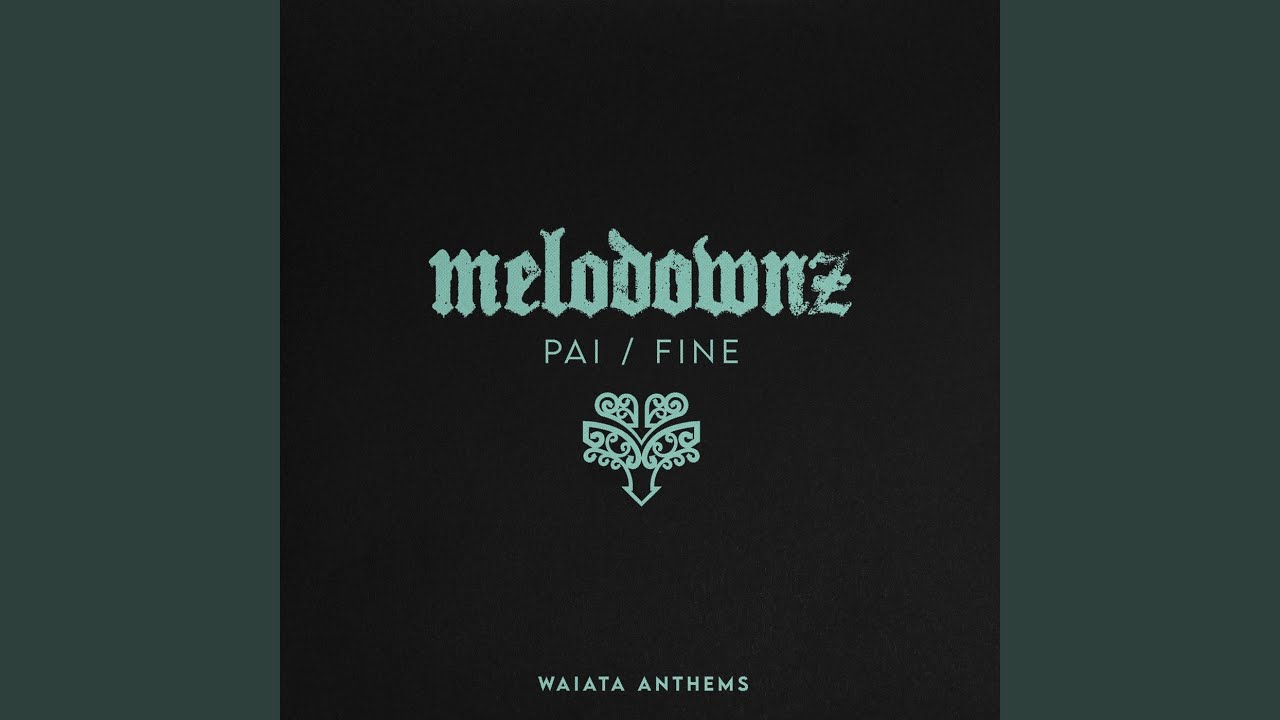The image resembles an album cover and is horizontally oriented. It features three primary panels: two vertically rectangular panels on the left and right in a muted dark green, flanking a central black square. In the center of the black square, there is white Gothic script that reads "Mellow Downz," with the 'Z' appearing slightly faded. Below this, in slightly smaller white letters, is the text "PAI/FINE" followed by a small emblem that looks like an abstract deer mask. At the very bottom, in small white letters, is the text "WAIATA Anthems." The overall style emphasizes graphic design typography.